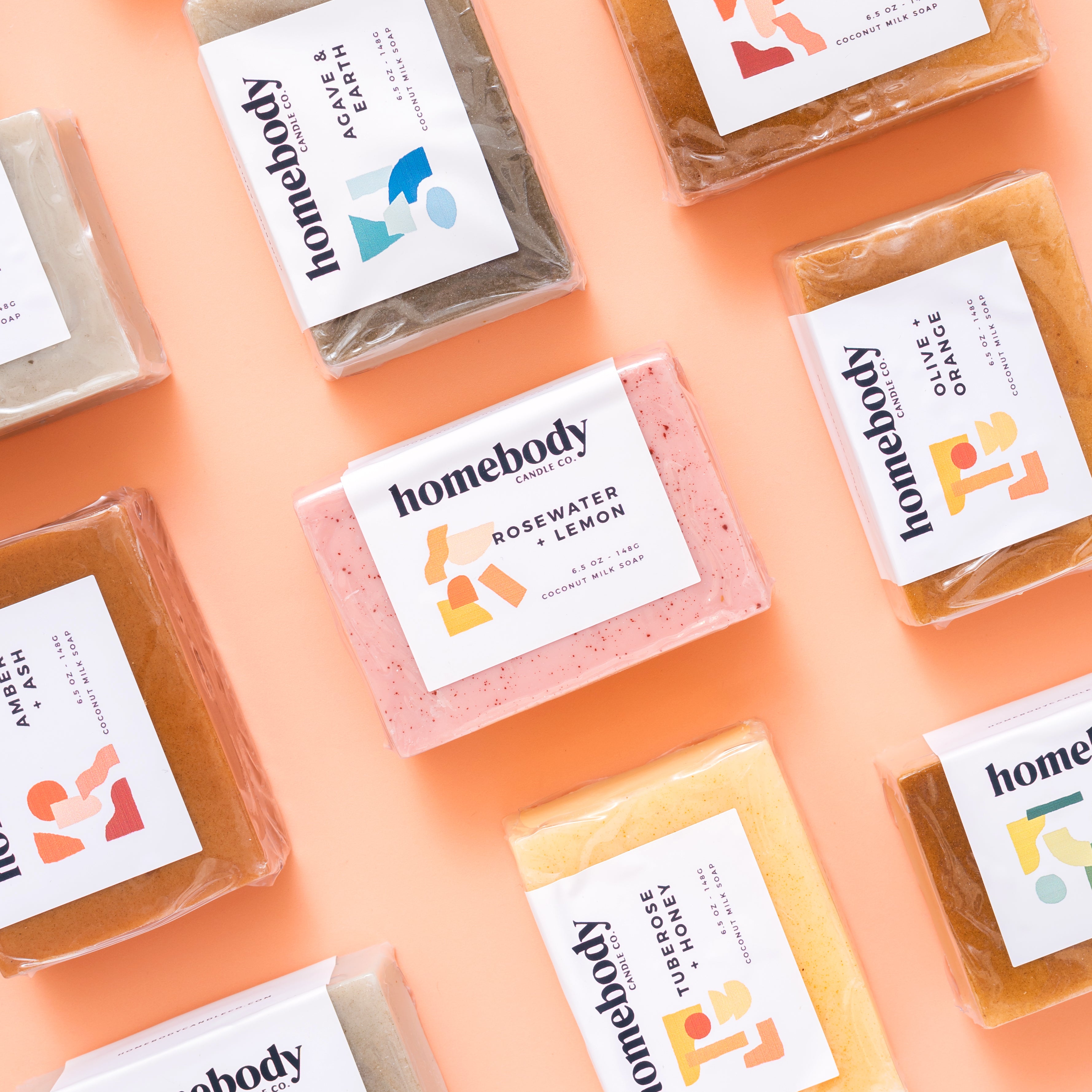This photograph showcases a beautiful array of handmade soaps meticulously arranged on a peach-colored surface. The brand name, "Home Body," proudly appears in bold black font at the top of each soap's packaging. Each soap is individually wrapped in plastic, reflecting light and adding a touch of elegance to the presentation.

Towards the bottom of the image, a peach-colored soap labeled "Tuberose and Honey" stands out with its soft hue. Adjacent to it, an orangey-tan soap marked "Olive and Orange" brings warmth to the collection. A slightly darker orange soap, named "Amber and Ash," adds depth to the display.

In the center, a captivating pink soap with red speckles, identified as "Rose Water and Lemon," draws the eye with its delicate coloration. Above it, a soap with a darker, grayish tone is partially visible, though the label is not fully readable.

While some soaps at the bottom are obscured and their labels cut off, the diverse scents and colors presented create an inviting and aromatic visual experience. This array of handmade soaps emanates a sense of artisanal craftsmanship and careful attention to detail.